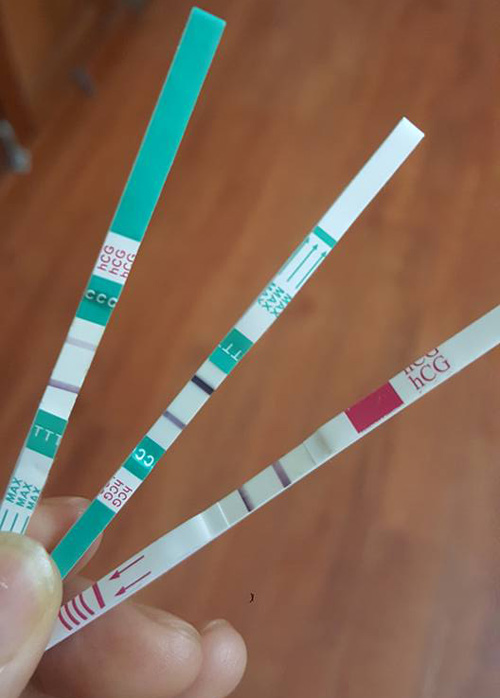A close-up image depicts a well-groomed, clean white hand, with four fingers visible, against a medium brownish-red wooden floor. The hand is holding three test strips, arranged similarly to Wolverine’s claws or a small rake. The strips measure approximately three to five inches in length.

The first strip, the widest, features a mix of green and white colors with text in varying orientations. It contains three sets of red letters "hCG," with the 'H' in lowercase and the 'C' and 'G' in uppercase. Horizontally across the strip are three green 'C's, interspersed with faint rust-red white lines. The strip further displays three white 'T' letters in a green square and is marked with the word 'MAX' in uppercase, flanked with green lines.

The second strip is slightly thinner and appears to be held upside down relative to the first. The third strip, devoid of green, is predominantly white and red. It also bears the "hCG" label in larger red text on a white background, a red square, and rust-hued middle lines. Additionally, it features two red diagonal left-pointing arrows and five red stripes, four of which are curved, while one is straight.

The arrangement of the strips and their similarities to test kits suggest that these may be diagnostic tools, akin to those used in COVID-19 or pregnancy tests.